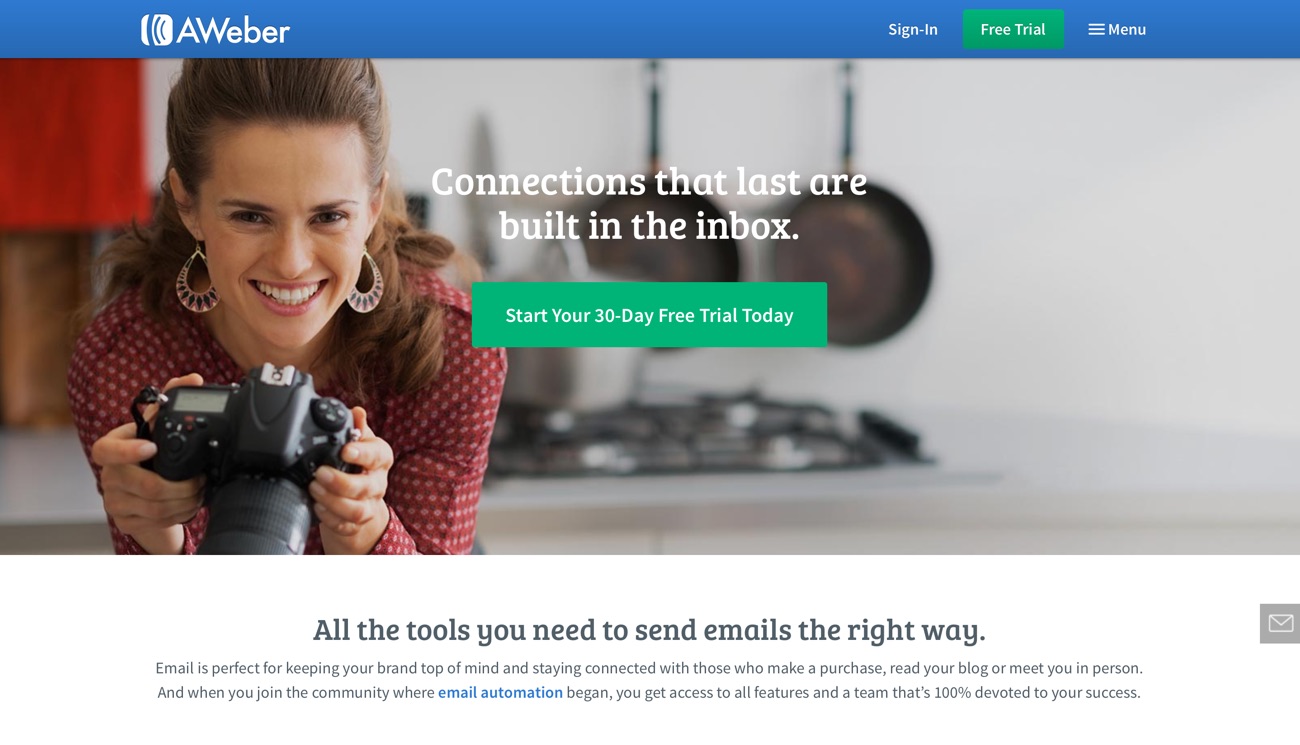The image displays a green bar across the top featuring a white logo. The logo includes a smaller white curving line beside a larger white curving bar with two blue curving lines inside it, accompanied by the text "A. Weber." To the right of the logo, there are options labeled "Sign In" and a green rectangular button that says "Free Trial." Additionally, a menu icon comprising three horizontal lines is visible, labeled with the word "Menu."

The central focus of the image is a photograph of a woman in a kitchen. She is wearing long earrings and a red printed dress. Behind her, kitchen pans are hanging in the background near a stove. The woman is holding a camera. Overlaying the image, the text reads, "Connections that last are built in the inbox."

Below the photograph, another green rectangular button prompts viewers with "Start your 30-day free trial today." Further down, in smaller text, it states, "All the tools you need to send emails the right way." There is additional text at the bottom, which is mainly in black with some lines in blue, though it is too small to be legibly detailed.

On the right-hand side, a gray rectangular box features a white outlined envelope icon.